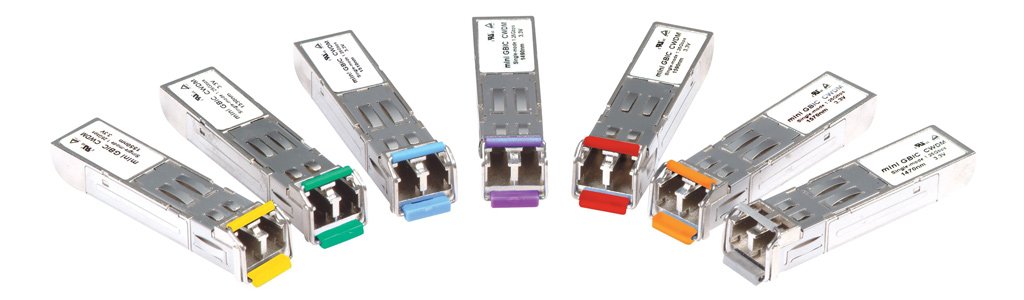This is a product photo set against an all-white background, featuring seven long rectangular prisms that resemble metal cages or containers. These objects, possibly tools or electronic components, are made of a metallic gray-silver material and are arranged in a semi-circle with their colored ends facing inward. Each prism has distinct, vibrant colors at their front tips: yellow, green, light blue, purple, red, orange, and gray, from left to right. Some models suggest they have openings with slots, and each one has a white sticker with three lines of black, illegible text on the top back end.